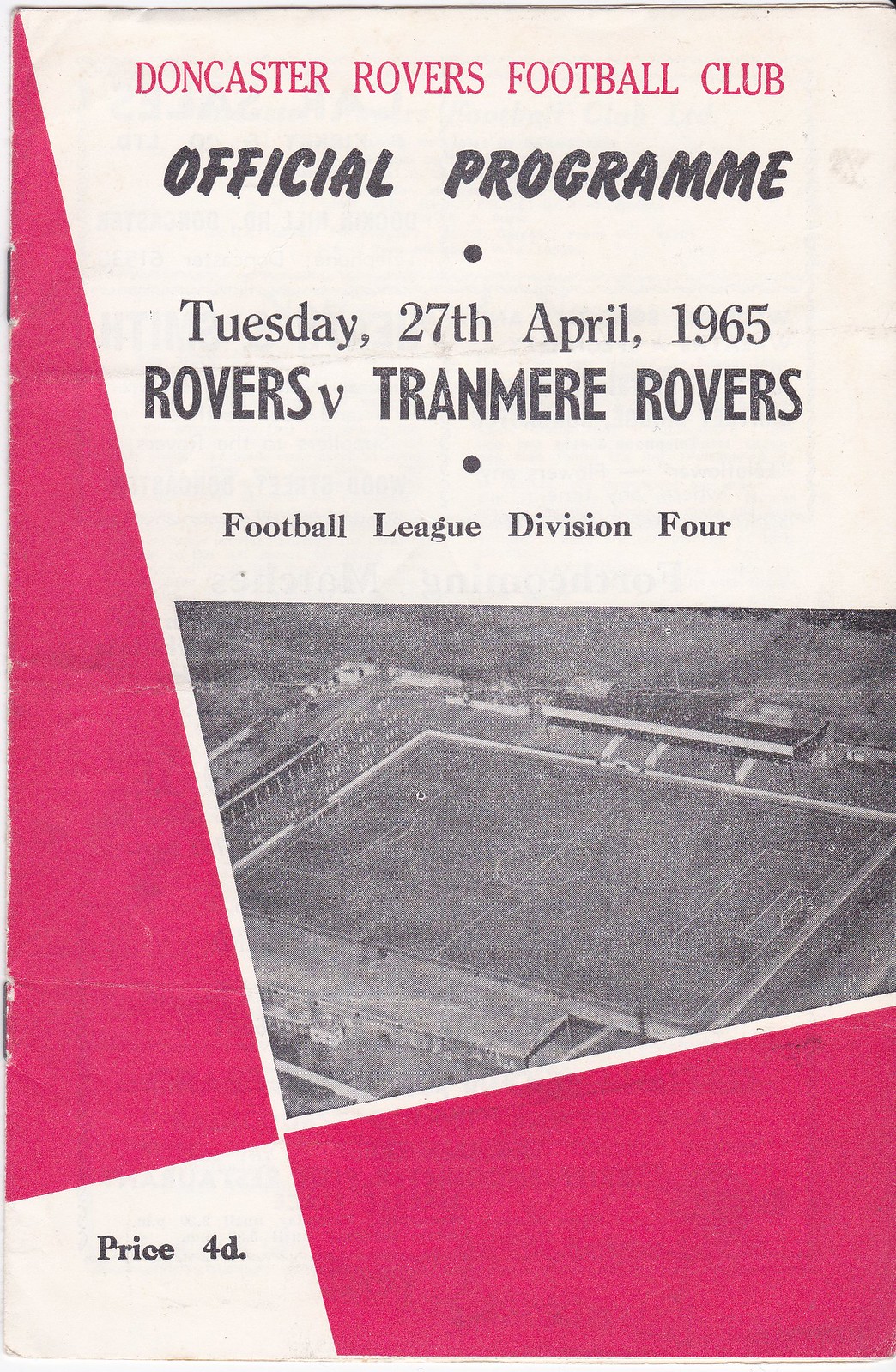The cover of this vintage football program from an English soccer game features the Doncaster Rovers Football Club. The program, dated Tuesday, 27th April 1965, is for a match between Doncaster Rovers and Tranmere Rovers in the Football League Division 4, priced at 4D. The design is geometrical with a primarily white background, accented by pink (or red) triangles and rectangular shapes that meet near the bottom left corner where "Price 4D" is inscribed. The title "Doncaster Rovers Football Club" is written in pink at the top, followed by "Official Program" and the match details in black font. Centrally, there is an aerial shot of a football field in black and white, adding to the vintage feel of the worn-out cover.